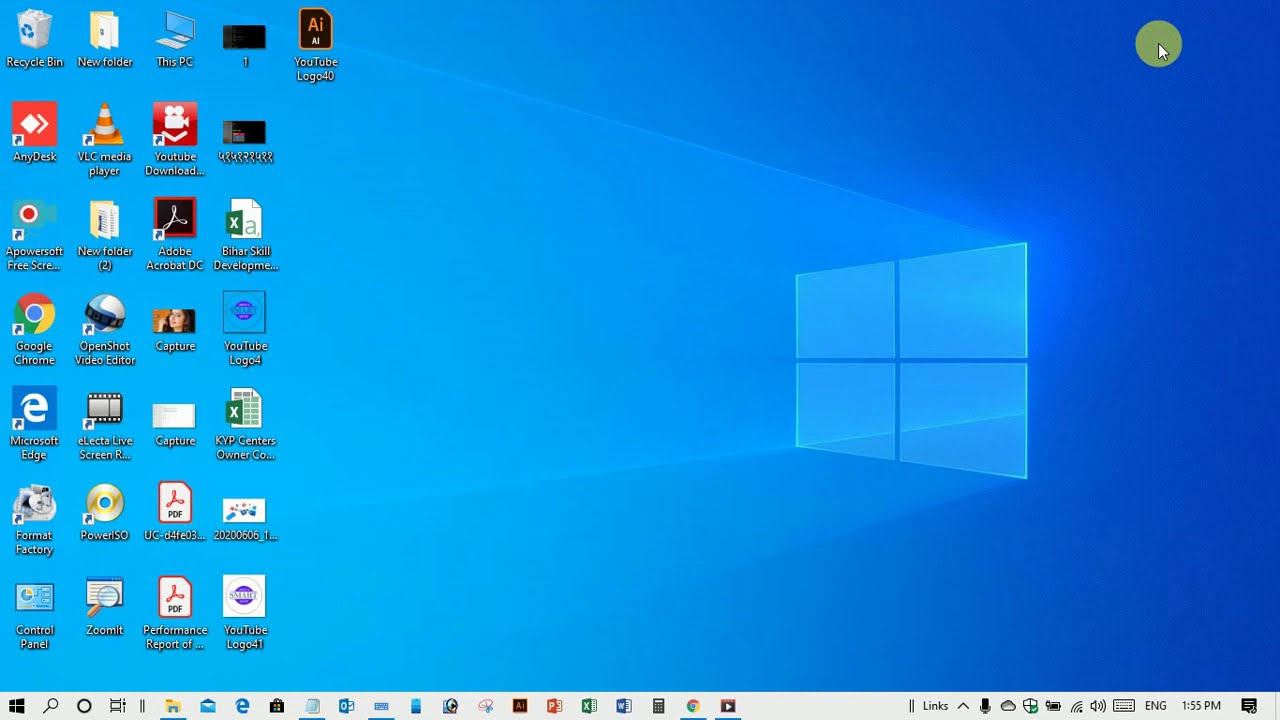The image depicts the desktop screen of a Windows computer with a blue background and the modern Windows 10 logo prominently featured towards the center-right of the screen, characterized by its cross and four sections design emitting a lighter blue glow from the Windows panes. The upper right-hand corner shows a cursor positioned within a yellow circle, indicating mouse activity. On the left-hand side of the screen, several standard icons are arranged in columns, including shortcuts for This PC, Google Chrome, Microsoft Edge, Recycle Bin, and other miscellaneous files such as PDFs, Adobe Illustrator files, Excel worksheets, and some new folders. The bottom taskbar includes the Windows logo, Internet Explorer, and other open applications, along with the usual system icons like the Wi-Fi symbol and the sound control. The timestamp in the bottom-right corner reads 1:55 p.m., suggesting the screenshot was taken in the afternoon.